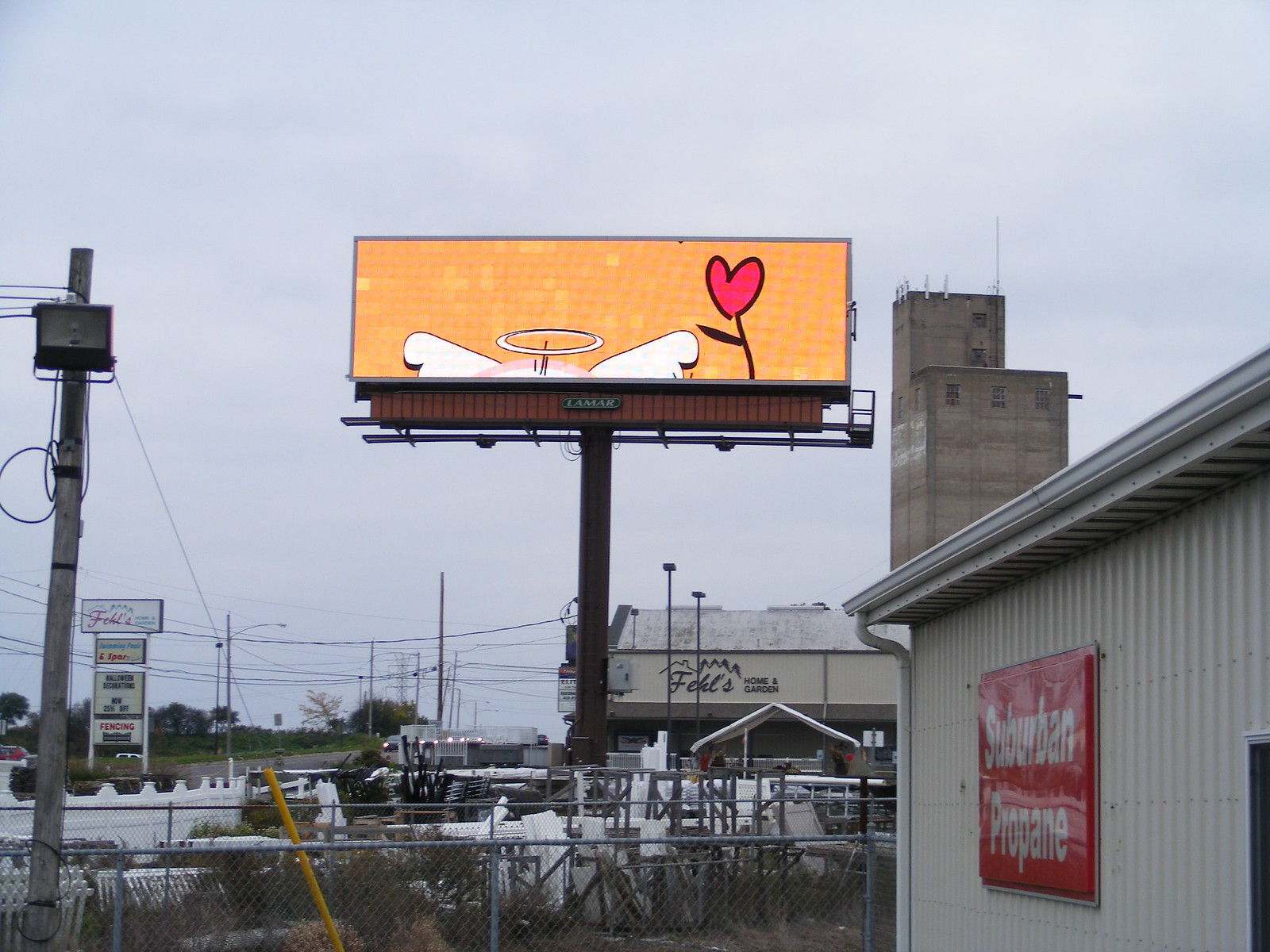This outdoor scene captures a bustling highway under a cloudy afternoon sky. Dominating the image is a prominent beige billboard featuring a heart-shaped flower design. Just visible at the top of the billboard is what appears to be the antenna and white ears of an alien-butterfly-like character, reminiscent of Hello Kitty. On the left side of the image, a collection of stacked signs points to a shopping strip with various businesses, although the specifics are unclear due to the distance. In the foreground to the right, a sign indicates the availability of propane, hinting at a nearby vendor. Additionally, a building that could be a school is partially visible further right. The scene is interspersed with typical street elements such as overhead wires and streetlights, completing the everyday atmosphere of this busy roadway.